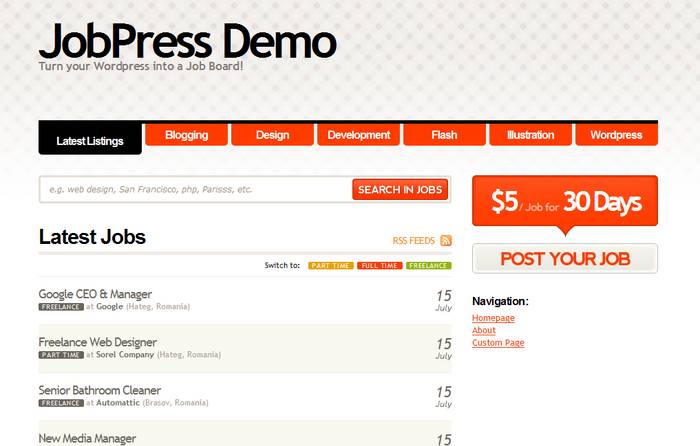The screenshot showcases a "Job Press Demo" website, designed to transform a WordPress site into a job board. Prominently displayed in the top left corner is the site branding with the tagline, "Turn your WordPress into a job board." The main navigation bar features multiple tabs, including "Latest Listings," "Blogging," "Design," "Development," "Flash," "Illustration," and "WordPress." The "Latest Listings" tab is currently active.

Beneath this tab is a search bar with placeholder text suggesting examples like "EG web design, San Francisco, PHP, Parisa, ETC." Adjacent to the search bar is an orange button labeled "Search in Jobs." The section below lists the most recent job postings, including positions for "Google CEO and Manager," "Freelance Web Designer (Part-Time)," "Senior Bathroom Cleaner (Freelance)," and a partially visible listing for a "New Media Manager."

On the right side of the page, there's a vivid orange rectangle offering a "$5 job for 30 days." Below this, a white rectangle with orange text invites users to "Post Your Job." Additional navigation links for "Home Page," "About," and "Custom Page" are also available.